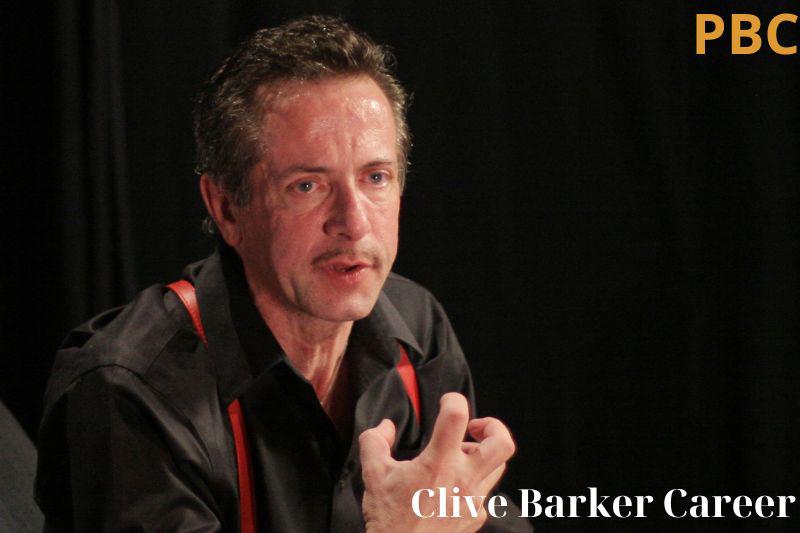The image captures a Caucasian man, identified by white text as Clive Barker, in the bottom right. The man, presumably Clive Barker, has short brown hair, blue-gray eyes, and a pencil-thin mustache. He appears to be animatedly speaking or explaining something, with his mouth slightly open and his right hand held up in a dramatic, claw-like gesture, as if emphasizing a point. He wears a black dress shirt, unbuttoned at the neck, and red suspenders featuring a red leopard pattern. The background consists of dark curtains, suggesting he is on a stage or in a similar setting. Additional text on the image includes "PBC" in yellow in the top right corner and "Clive Barker Career" in white at the bottom right. Clive Barker's face shows visible lines, indicating his older age, and he gazes off into the distance.